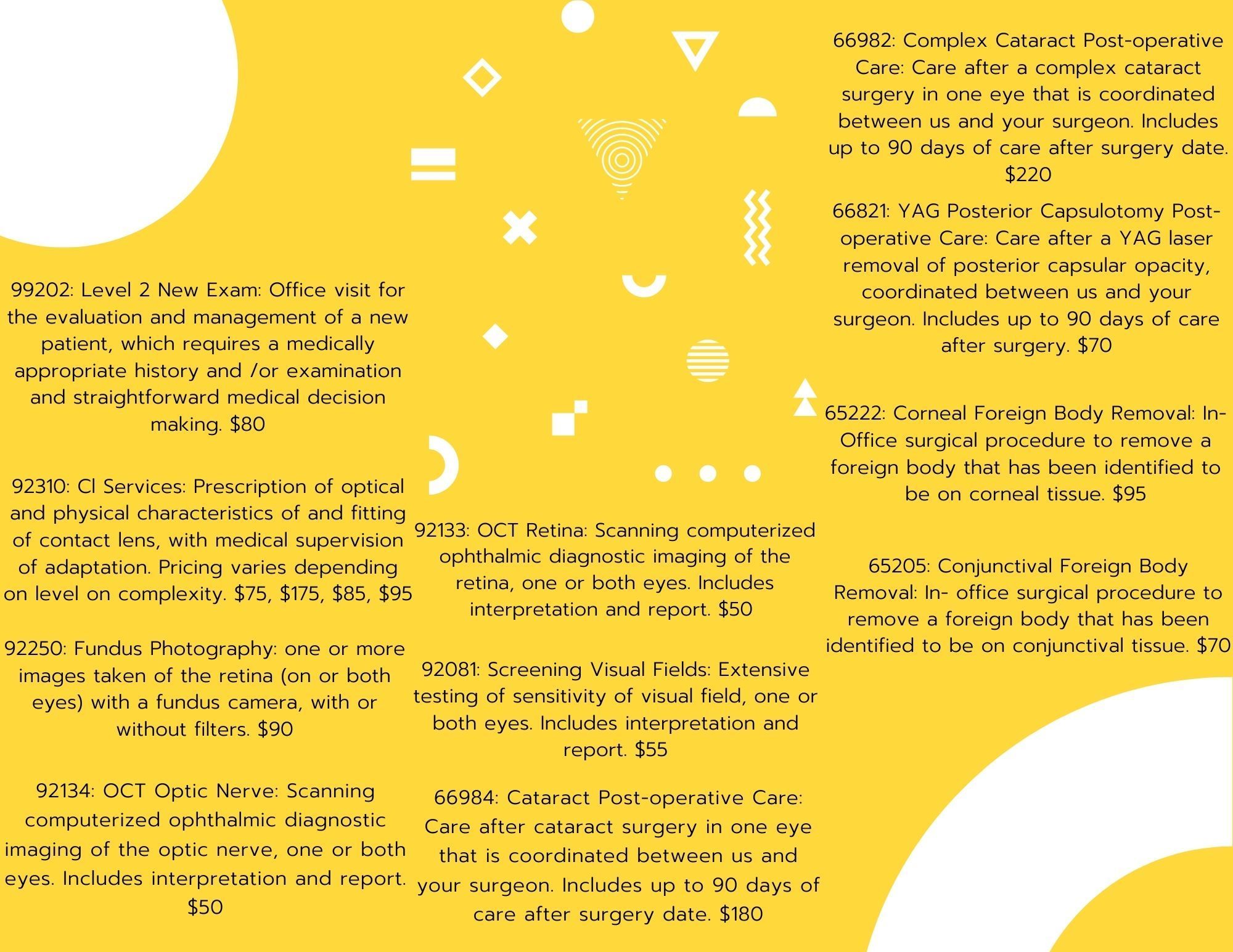The image is of a detailed price sheet for various eye care procedures, likely from a medical office or optometrist. The background is a light orange or mustard yellow, adorned with white geometric shapes, including triangles, semicircles, X patterns, inverted triangles, and squiggly lines. The text on the poster is predominantly in blue and contains numerous sections, each about a paragraph long. Each section pertains to different medical procedures, such as corneal foreign body removal, new patient examinations, contact lens fittings, and postoperative care for cataract surgery or YAG laser treatments, complete with prices and procedure codes like 99202 and 92301. Prices vary depending on the procedure and complexity; for example, a new patient evaluation (99202) costs $80, while the care following a complex cataract surgery (66982) and YAG laser treatment (22066821) posts a price of $70. There are 11 such entries listed on the poster, giving it the appearance of a proverbial menu of medical operations with accompanying costs.